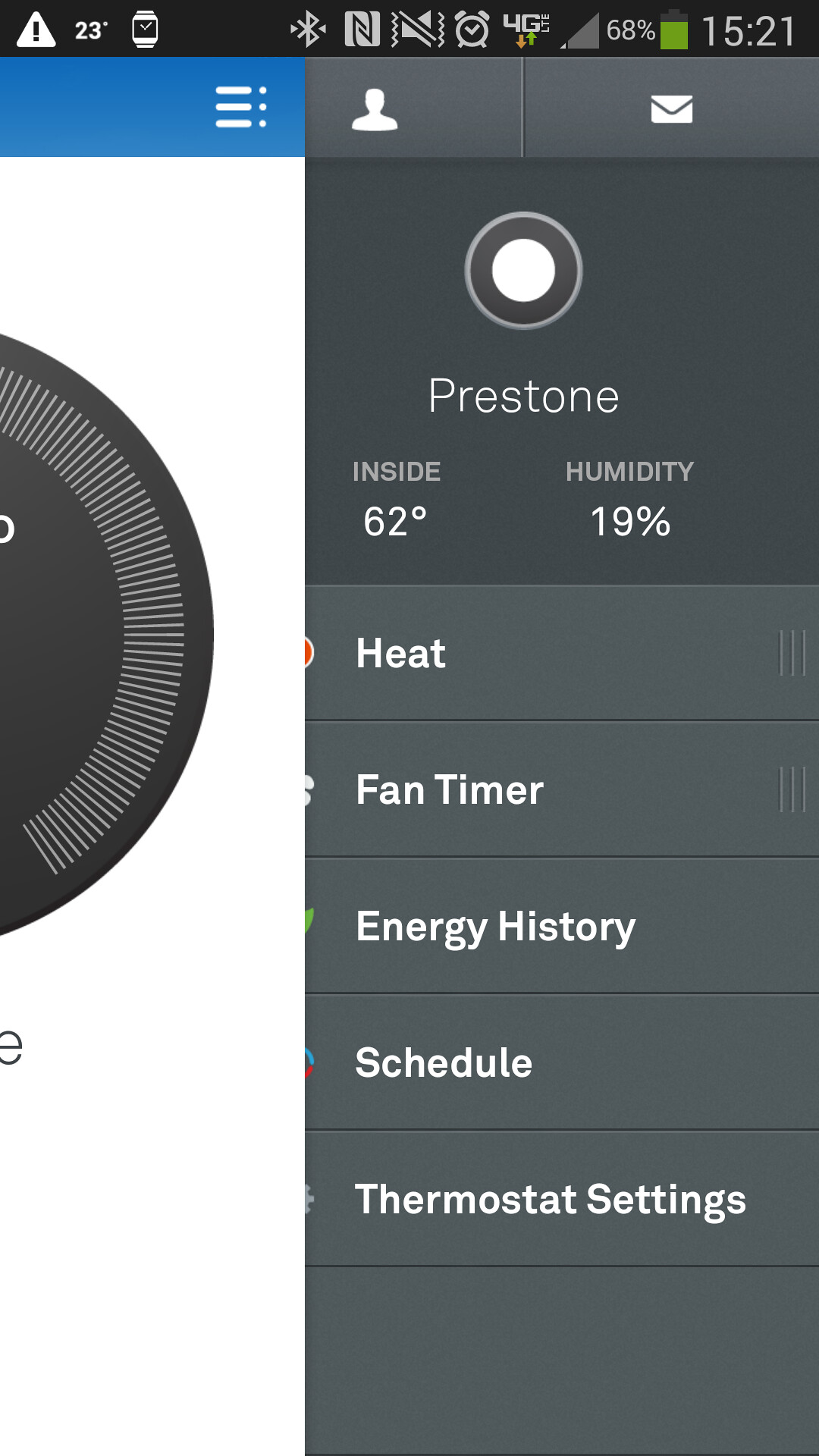This image appears to be a screenshot taken from a cell phone, displaying the control interface of a digital thermostat app. The status bar at the top features several icons in white font: an exclamation mark followed by "23", a watch-like icon, a silenced phone icon with a slash through the volume area, a clock icon, a 4G signal indicator accompanied by orange and green arrows, and a battery icon showing 68% charge with some green coloring. Adjacent to the battery icon, it reads "15:21".

The main screen of the app is divided into two sections. On the left side, against a dark gray background, there are several white icons and texts: a head and shoulders icon, an envelope icon, and a white circle labeled "Prestone." Inside the circle, the temperature reads "62°F" and the humidity is "19%". Below these, there are menu options labeled "Heat," "Fan Timer," "Energy History," "Schedule," and "Thermostat Settings."

On the right side of the image, there is a large black circle with white dash marks, set against a white background. Above this circle, a small blue bar appears with text that resembles lined notebook paper and includes three dots next to it, indicating additional options or a menu.